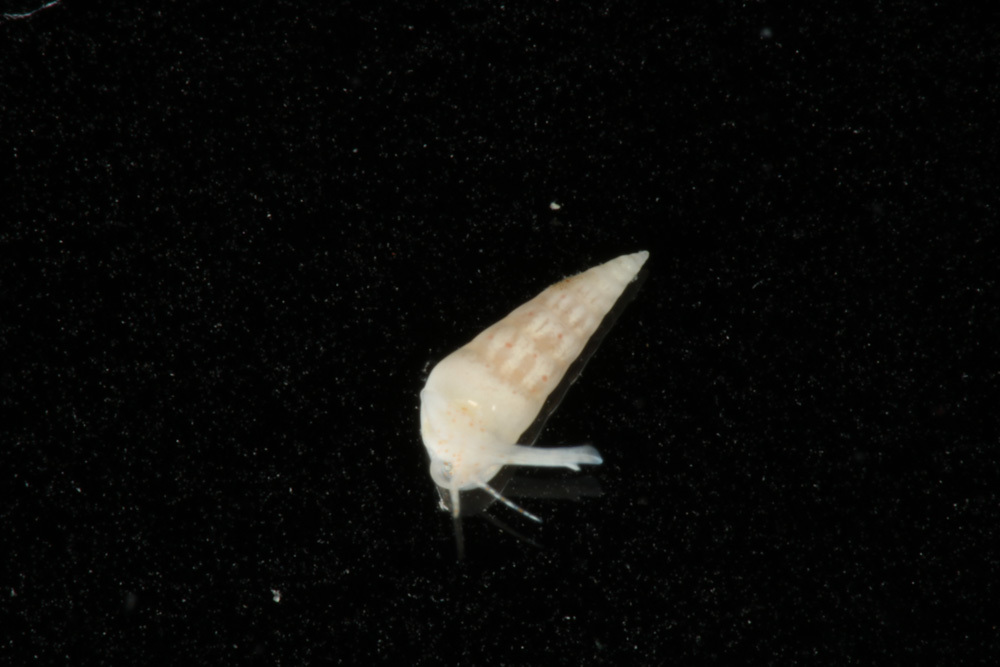The image is a high-contrast photograph featuring a small, snail-like creature, centrally positioned against a deep black and speckled background. The creature, called a rhizonia, has a creamy white, triangular cone-shaped shell with intricate patterns and light brown shading near the end, which tapers to a sharp point. The surface below reflects this rhizonia, adding a sense of depth, and is sprinkled with various sized white specks. Red dots adorn the recessed areas of its shell, providing a striking contrast. The rhizonia appears bulbous towards the front with a visible appendage or head extending towards the bottom right corner. Additionally, the creature displays a series of antennae and legs, accentuating its insect-like appearance amidst the reflective black backdrop.